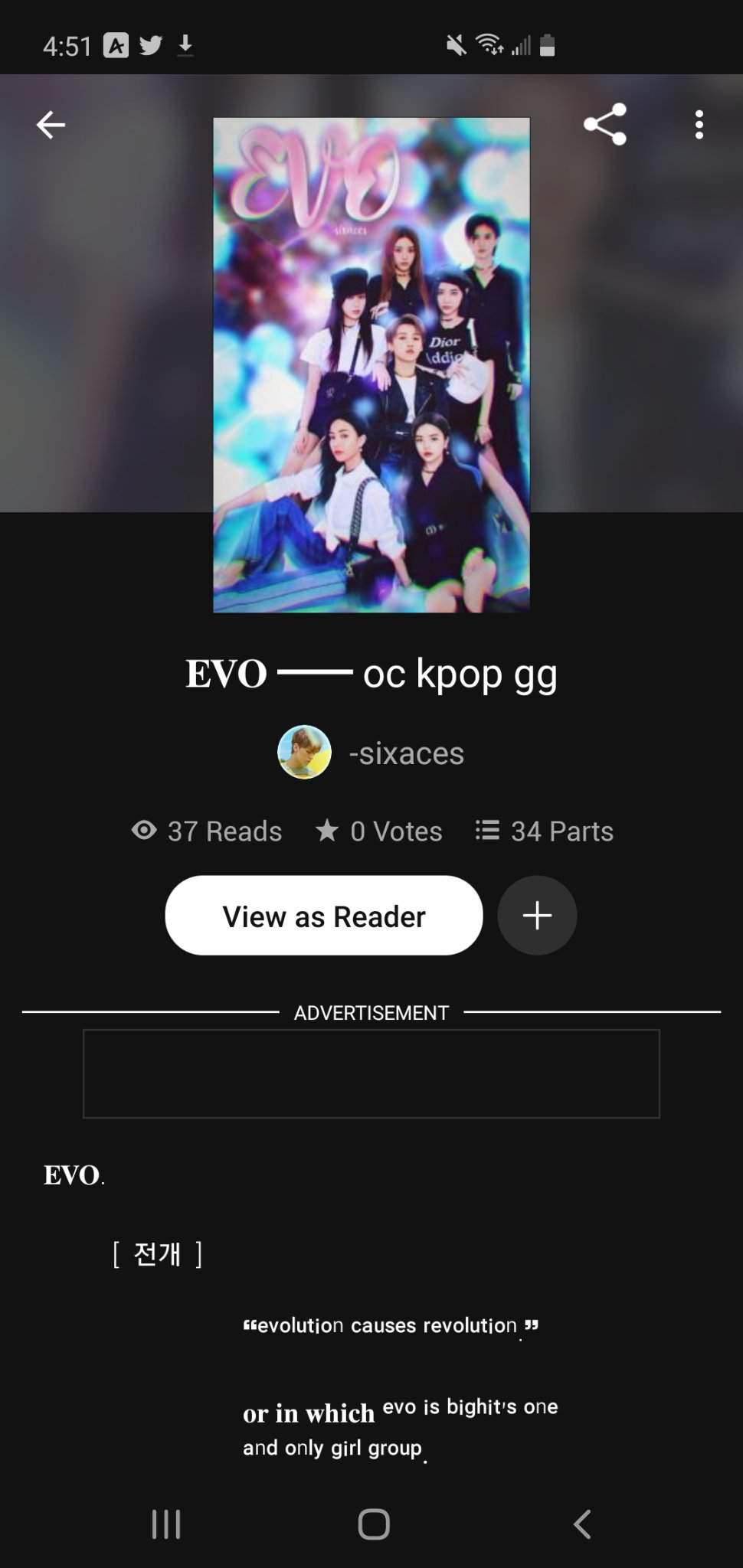This screenshot captures a vibrant section of a K-pop website. Dominating the top of the screen is a striking poster featuring the name "Evo" or "Eve," stylized in bright pink text against a dynamic background, positioned prominently in the top left corner. The centerpiece of the poster is a group photo showcasing a K-pop ensemble. The group appears to consist of six or seven members, including a mix of females and one or two males. The posing arrangement is casual yet coordinated, with two members seated on the ground and another huddled closely with the rest, creating an intimate and cohesive snapshot.

Directly below the poster, bold text reiterates the name "Evo," followed by a line of text displaying "OC, K-pop, GG," possibly indicating the genre or categories related to the group or content. Just beneath this, a small, circular profile picture accompanies the username "Dash" with the subtitle "Six Aces." Further textual details reveal the website’s engagement metrics for this particular content: "37 Reads," "0 Votes," and "34 Parts," suggesting segmented content or a series. At the bottom of this section, a pill-shaped button labeled "View as Reader" invites users to experience the content in a reader-friendly format. The overall layout and vivid visuals emphasize the dynamic and engaging nature of the K-pop community featured on this site.